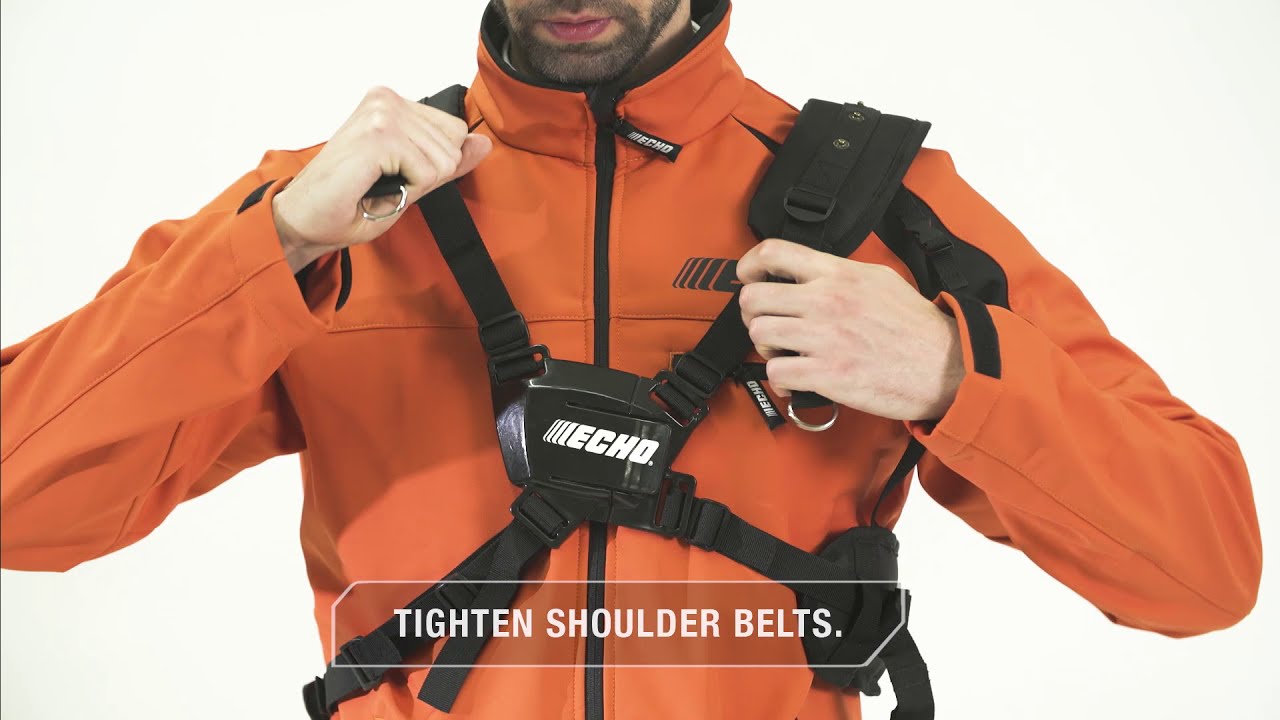The image features a detailed advertisement for sports gear, potentially for skydiving, centered on a Caucasian man wearing a bright orange jacket with black trim and a black zipper. The image focuses on his upper body, from just below his nose to his mid-torso, emphasizing his short, stubby brown beard and pink lips. The man is equipped with a black harness, featuring the word "ECHO" in white font at its central connecting point. His hands are gripping the shoulder straps, appearing to tighten them, aligning with the white text overlay at the bottom of the image that instructs, "Tighten Shoulder Belts." The background is completely white, making the man and his gear the central focus, underlining the instructional or promotional nature of the image.